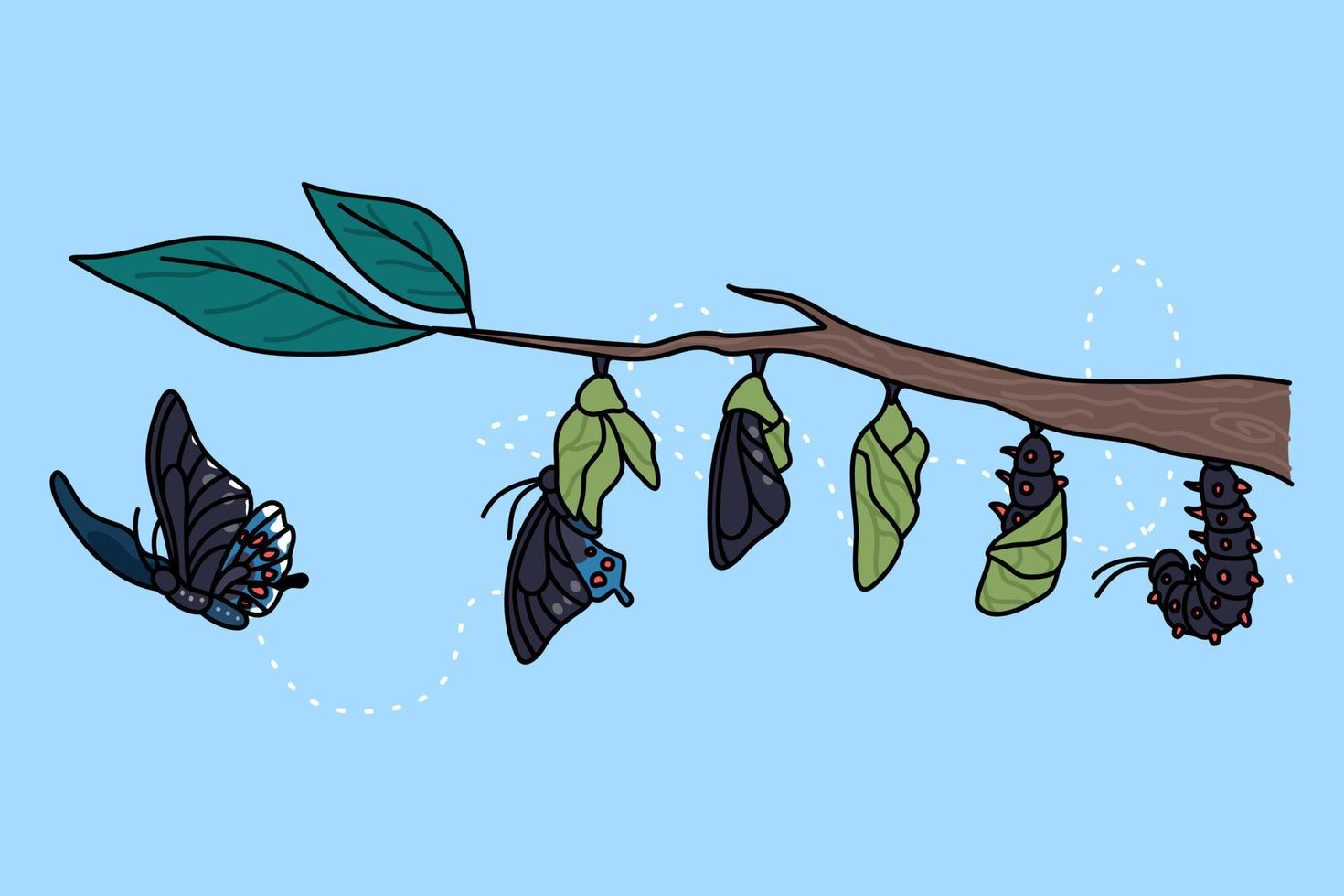The image is a cartoon-like, color illustration with simple black outlines and a pale baby blue background. It depicts the stages of butterfly metamorphosis on a thin tree branch, which extends from the right side of the image and has two pointed green leaves at the tip. Starting from the right side of the branch, there is a caterpillar attached by its rear end. Next, there is a caterpillar beginning to spin its cocoon, followed by a completely enclosed chrysalis. Subsequently, there is a chrysalis with butterfly wings emerging from it, followed by a butterfly sitting atop the open cocoon drying its wings. Finally, to the far left, a fully developed blue-gray swallowtail butterfly with white and orange spots is shown flying away. Dotted lines trace the butterfly's path from the cocoon to its current position in flight.